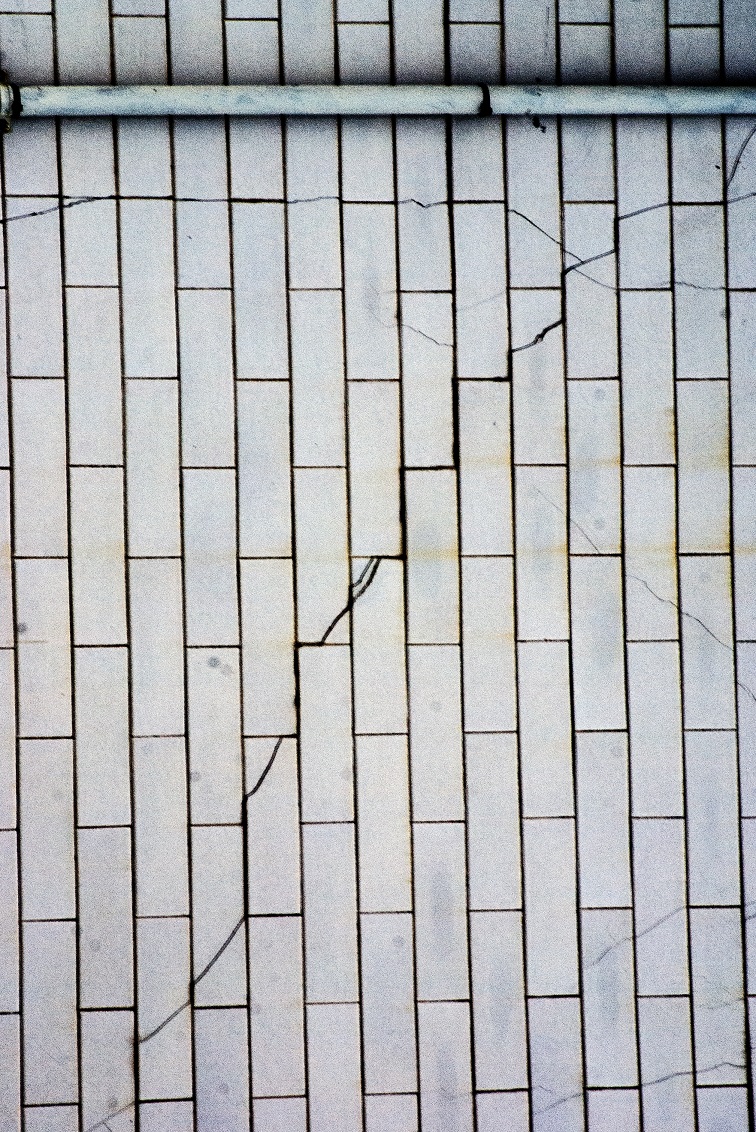The image is a rectangular photograph of a weathered and old tiled wall, resembling exterior brickwork. The tiles are long and rectangular, similar in length to bricks but slightly slimmer, and they are arranged in a staggered vertical pattern. The tiles themselves are white but exhibit significant discoloration, with some tiles showing greyish hues, yellowing spots, and dingy orange rust marks. The grout between the tiles is either black or heavily soiled, adding to the aged appearance. Cracks permeate the wall in various directions: diagonally from the bottom left to the top right, horizontally near the top, and vertically. Additionally, there's a whitish-grey pipe attached to the wall a bit down from the top, held in place by two straps, which also shows signs of age and markings.